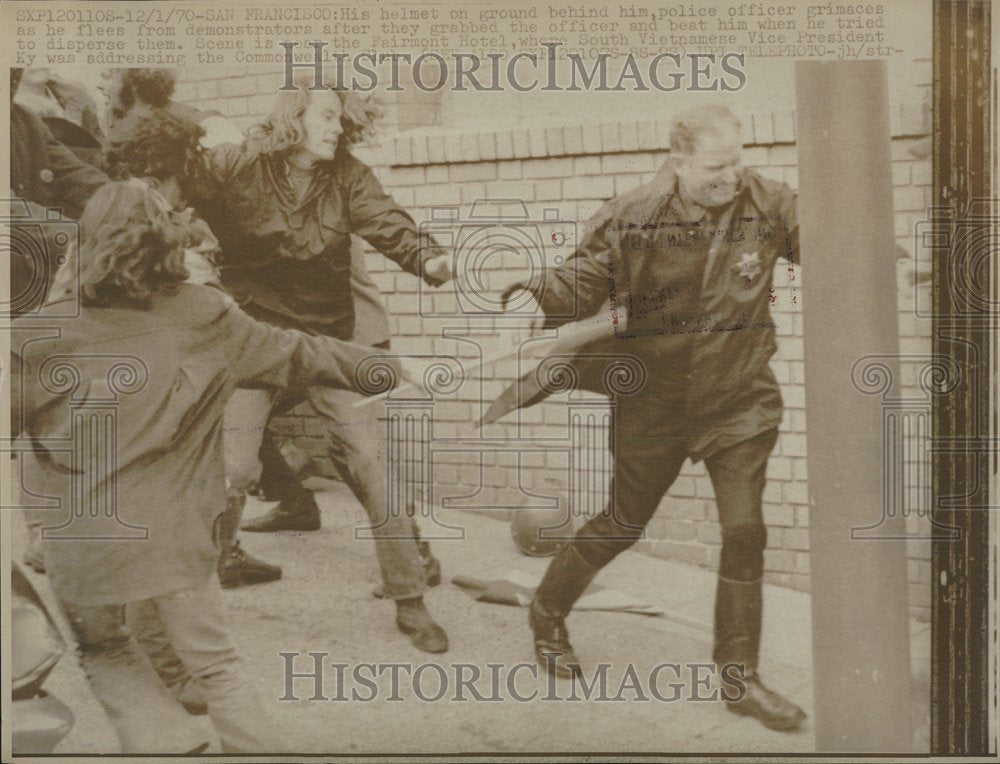The image is a sepia-toned, historic photograph depicting a chaotic scene in San Francisco, as detailed by the faded text "12-170 San Francisco" at the top. The central figure in the photograph is a Caucasian police officer dressed in a dark uniform with a visible sheriff's star on his jacket. He is depicted grimacing and fleeing to the right side of the frame, leaving his helmet on the ground behind him. The officer is being pursued by an angry mob of long-haired men, one of whom is jabbing him with a stick, while others appear to be trying to hold the officer back. The scene takes place on a sidewalk bordered by a brick wall. This unrestful moment is framed by a vertical wooden frame on the right edge of the image. Watermarks with the text "Historic Images" are prominently placed at the top and bottom center, with a large, transparent logo featuring "HI" and a camera in the center that spans the entire photograph. The dimensions of this rectangular image are approximately 5 to 6 inches wide and 4 to 5 inches high.